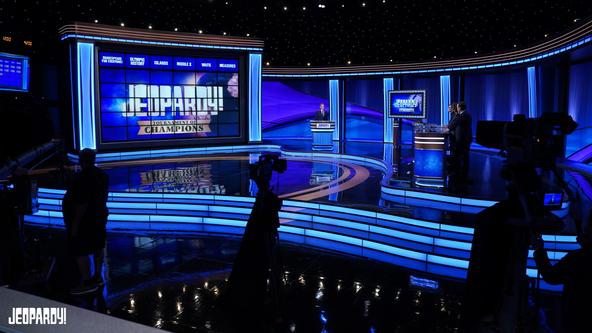The image captures the Jeopardy! stage from the audience's perspective. Prominently on the left side is the Jeopardy! board, with multiple screens displaying questions and answers. At the center of the board, "Jeopardy!" is emblazoned in large white letters. Below this, a gold-colored banner with some unreadable black text spans the width, while light blue columns flank the sides and a brown column runs along the top, with another light blue column at the bottom.

Dominating the middle of the stage is a podium from which the host operates, though he appears distant and indistinct. The podium features a blue lower part and a brown upper part with a white square, and to its right, there is another monitor with a blue background displaying "Jeopardy!". Beyond the host's podium, the contestants' black podiums are aligned, making the one in the forefront indistinguishable from the others.

The stage backdrop is a dynamic tableau of glowing blue and purple waves, creating an atmospheric contrast against the pitch-black ceiling, which is accented with lights along the edges. In front of the stage, silhouettes of audience members and large video cameras are visible, with a silhouetted camera operator positioned on the left. The floor in front of the stage is dark black, with yellow lights reflecting off its surface, adding to the luminescence and drama of the scene. The entire setup exudes the thrilling and competitive ambiance of a Jeopardy! Champions edition recording.